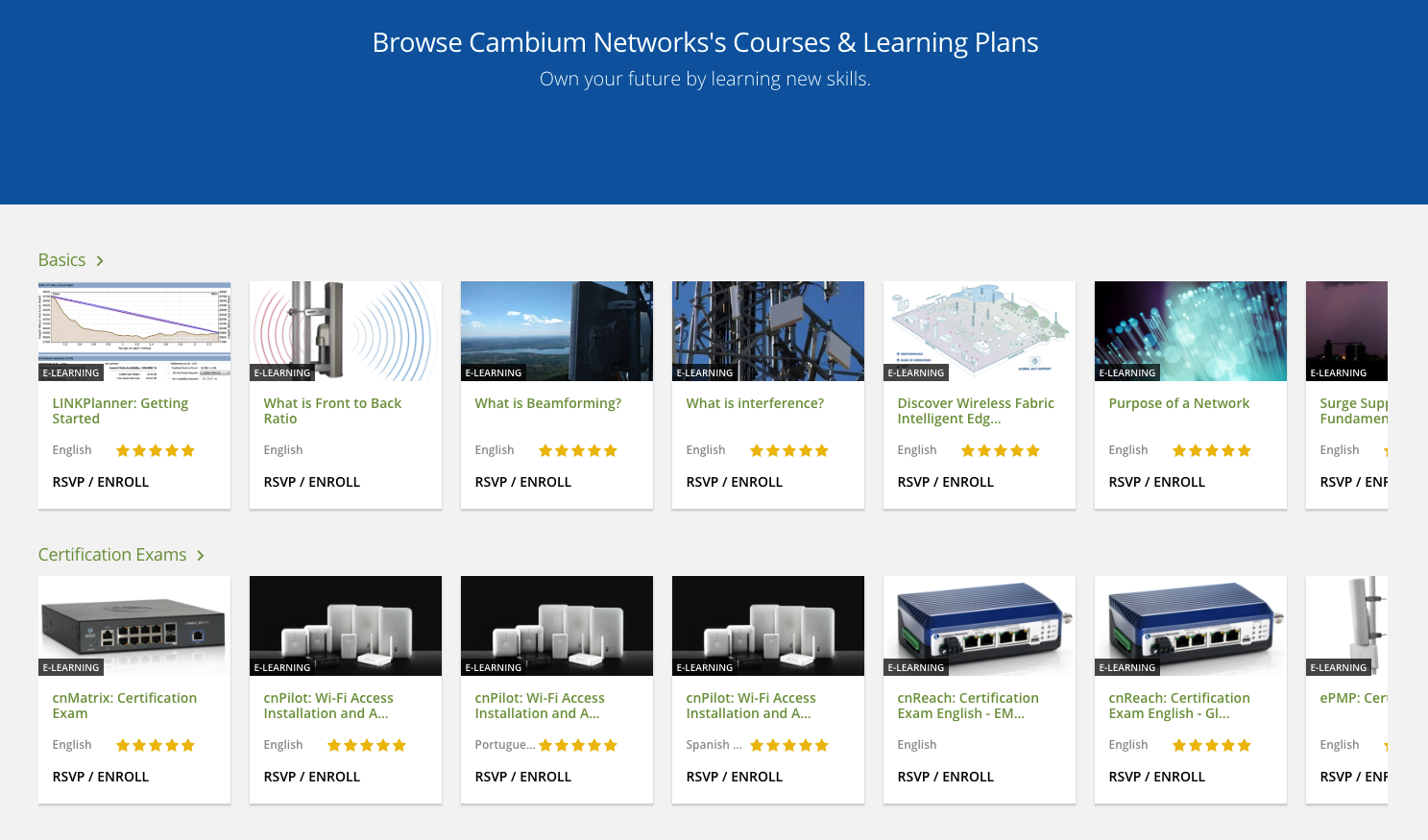This screenshot captures the webpage of an online learning platform, presenting a design reminiscent of Facebook's familiar blue and white color scheme. The top one-third of the page features a prominent blue banner, which spans the entire width and bears the message "Browse Cambium Networks Courses and Learning Plans" in bold white letters. Just beneath this title, a smaller white subtitle reads, "Own Your Future by Learning New Skills."

The remaining two-thirds of the page transitions to a clean white background. This area is divided into two rows, showcasing various courses and learning plans available for purchase, neatly organized and ready for user exploration. The layout and color scheme not only provide a sense of familiarity but also ensure an organized and aesthetically pleasing browsing experience.